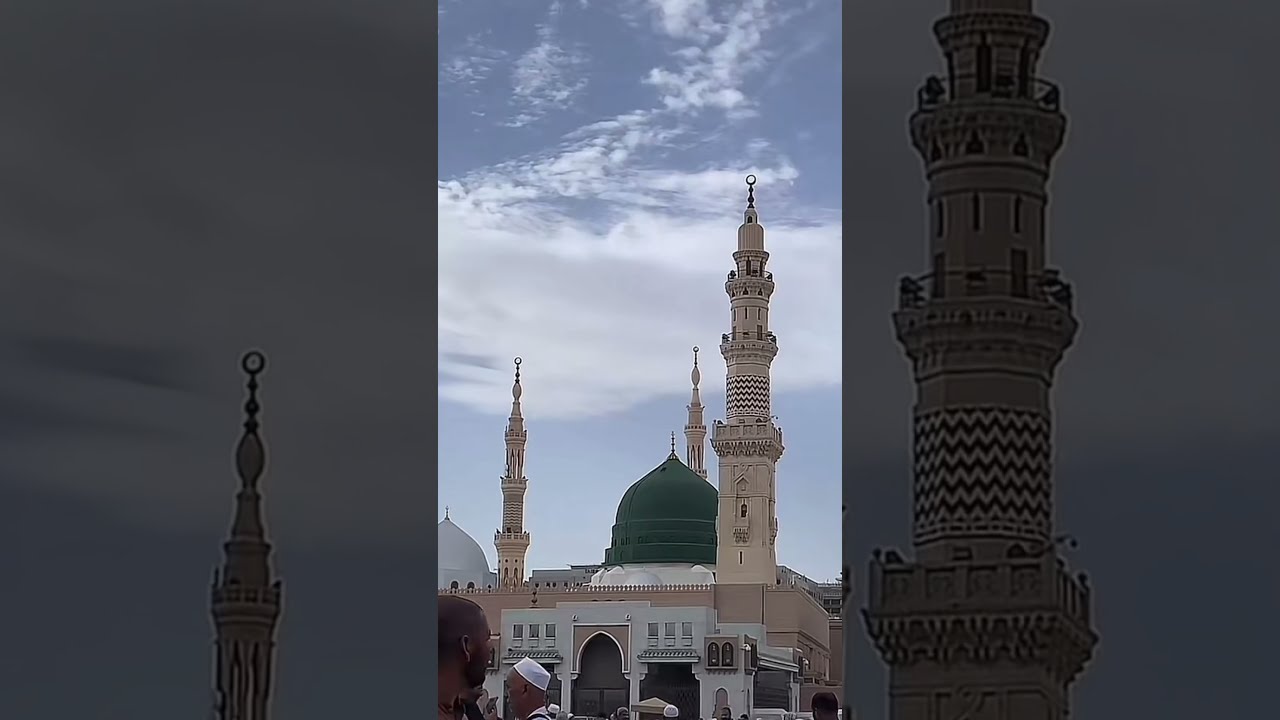The image is presented in three vertical sections: the outer sections are darkened, close-up shots of the central photograph. The central image depicts a grand mosque with a cream-colored facade and a large, centrally located dark green dome. Flanking the dome are three slender towers, or minarets, positioned at the rear, left, and right corners of the structure. The mosque is ornately designed and significant in scale. Below the architectural marvel, a number of individuals are visible, though only their heads are shown, some adorned with white caps indicative of traditional attire. The sky above is a vivid blue, embellished with a blanket of white clouds in the middle and wispier clouds toward the top, forming a striking backdrop. The outer sections provide a darker, zoomed-in view of the mosque’s towers, offering a detailed contrast to the brightly lit central picture.